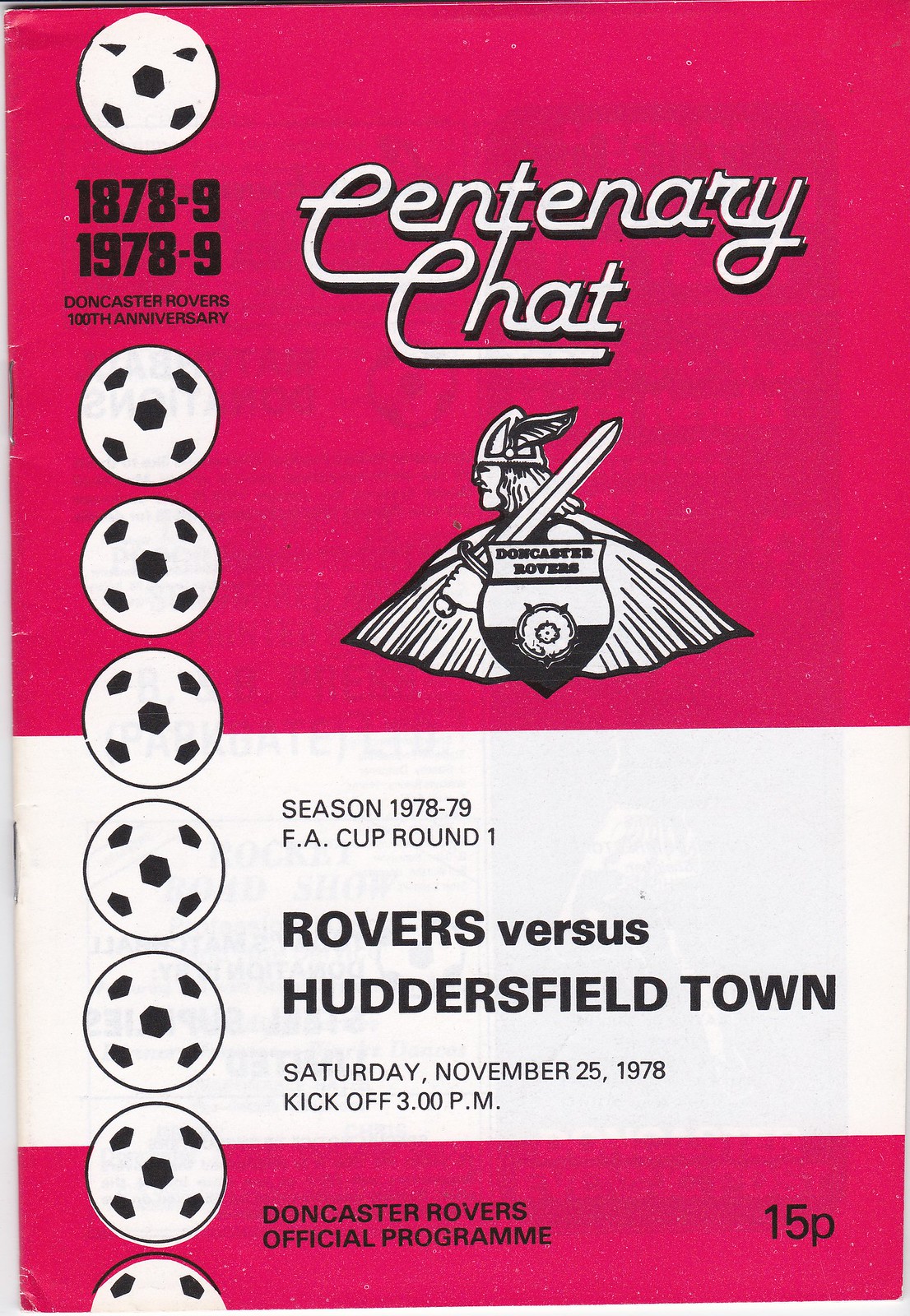The image is the cover design of a Doncaster Rovers official program celebrating their 100th anniversary. The cover features a red and white color scheme, with a white section flanked by red at the top and bottom. The top left corner displays the years 1878-9 and 1978-9, marking the centenary celebration. Along the left side of the cover, there is a column of eight soccer balls, with the anniversary years in place of the second ball. Prominently in the center-right, "Centenary Chat" is written in white cursive text with a black border. Below this, the Doncaster Rovers logo is depicted as a Viking with a flowing cape, a conical helmet with a wing, carrying a sword on his shoulder, and a shield that reads "Doncaster Rovers." The middle of the cover provides details of the event: "Season 1978-79, FA Cup Round 1, Rovers vs. Huddersfield Town, Saturday, November 25, 1978, kickoff 3 pm." The bottom red section notes this is the "Doncaster Rovers official program," priced at 15p. The entire cover appears as a scanned image, visible from the staples on the side.